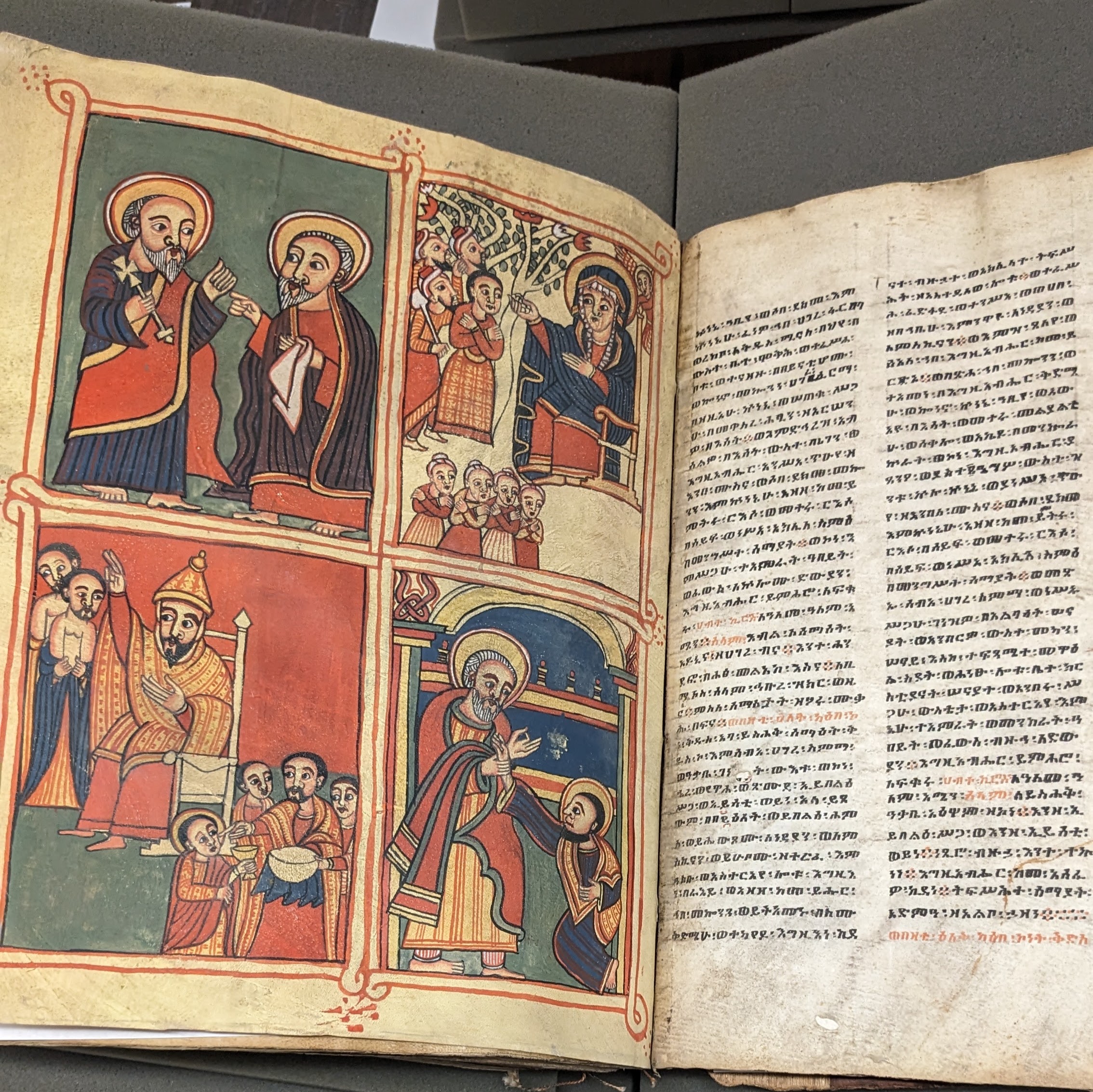The image depicts a meticulously preserved illuminated manuscript from the medieval period, set against a soft, grayish foam surface. The manuscript is open, revealing a page layout divided into two distinct sections: the left page adorned with four vibrantly colored vignettes, and the right page filled with foreign text.

The left side features four detailed illustrations arranged in a grid. The top left vignette shows two elderly men engaged in conversation, with one holding a cross, suggesting a religious context. The top right vignette portrays a king or high-ranking figure seated on a throne, surrounded by attendants who have their arms crossed. The bottom left vignette depicts a figure in an elaborate orange and yellow hat and garb, seated and addressing a group of children and adults. The bottom right vignette presents a man in orange, green, and yellow robes, with white hair, standing before a kneeling figure, holding the kneeler's hand in a gesture of blessing or supplication.

The right page comprises densely packed black text with certain sections highlighted in orange, perhaps to emphasize particular words or phrases. The text is foreign and unfamiliar. The manuscript's background is a beige material, likely parchment or vellum, indicating its antiquity. The colors in the illustrations are rich shades of greens, reds, browns, and blues, all outlined in black, though there is no gold present.

The manuscript is displayed in an environment that could be a library or museum, hinting at its historical and cultural significance. The overall condition is remarkable, considering its age, making it a precious artifact from a bygone era.